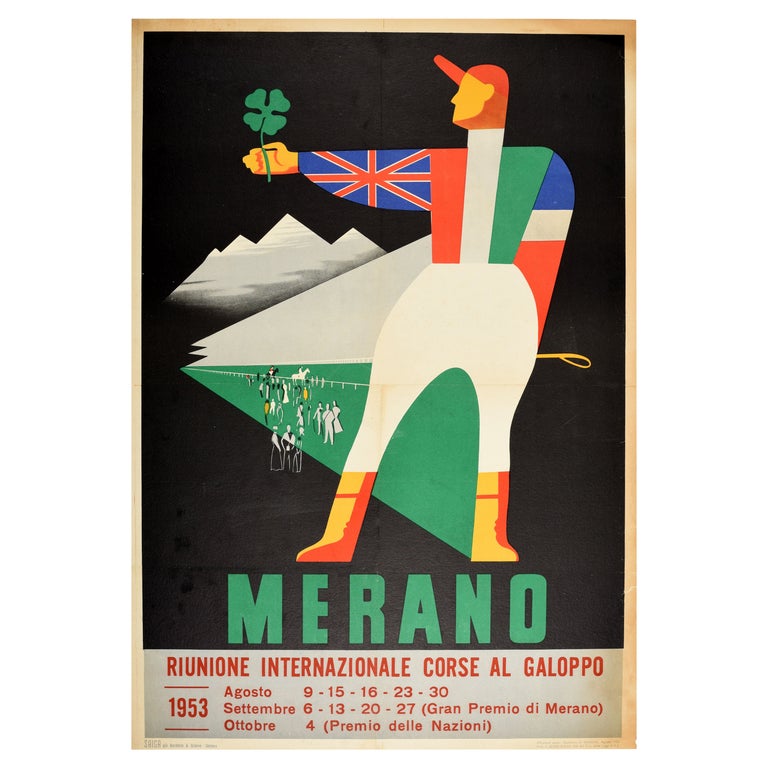This image is a detailed poster from 1953 advertising an international event, possibly horse racing, as indicated by the text and figures. The central figure is a stylized, colorful silhouette of a man dressed as a jockey. His face is not visible as he is turned to the left, extending his right arm to the side, holding a green four-leaf clover with a yellow hand. His attire is quite distinctive: the right sleeve features the Union Jack (British flag), while the chest section of the shirt is divided into three vertical sections of red, white, and green, resembling the Irish flag. The left sleeve appears to bear the pattern of the French flag. He wears white pants with exaggerated hips and orange boots. The background of the poster is black, adorned with a subtle white mountain silhouette and miniature figures of people and horses on a green field, suggesting a racecourse scene. The poster is bordered with an aged cream color. At the bottom, in green font, it reads "Murano," followed by "M-E-R-A-N-O" and "R-I-U-N-I-O-N-E," along with further details about the event "International Course El Galapo, 1953" highlighting various dates in August, September, and October.